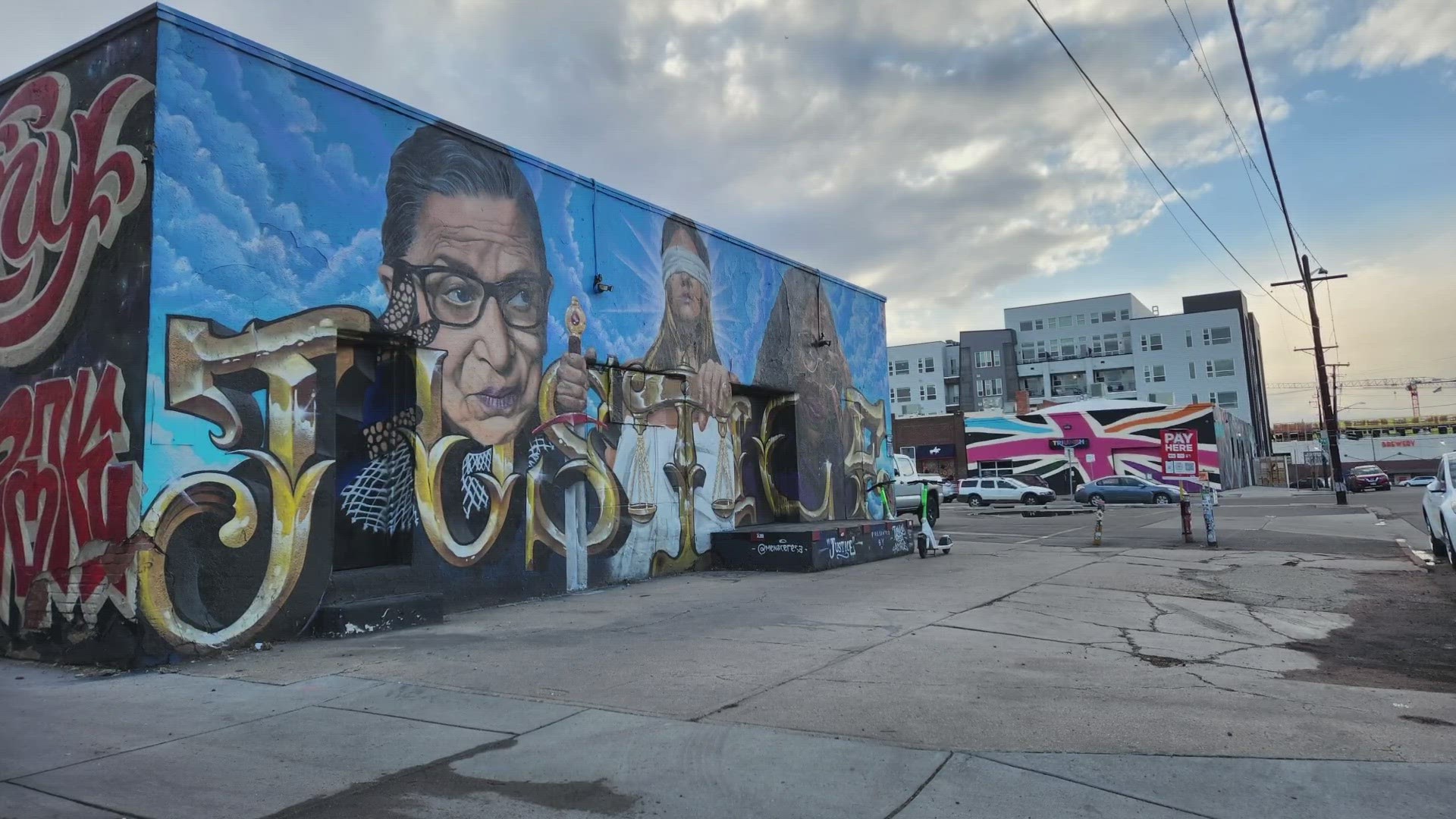The image captures a vibrant mural painted on the side of a building. The mural prominently features three figures, with Ruth Bader Ginsburg depicted first. Beside her, an image of a blindfolded Lady Justice holds her scales. The third figure is indistinct and unidentifiable. Spanning across the entire mural are the letters forming the word "Justice," rendered in an elegant gold font that stands out boldly against the background. The building with the mural faces a sidewalk, and in the background, a street and an additional apartment building are visible. The mural’s striking artwork is the focal point, dominating the composition and adding a sense of civic reverence to the urban landscape.